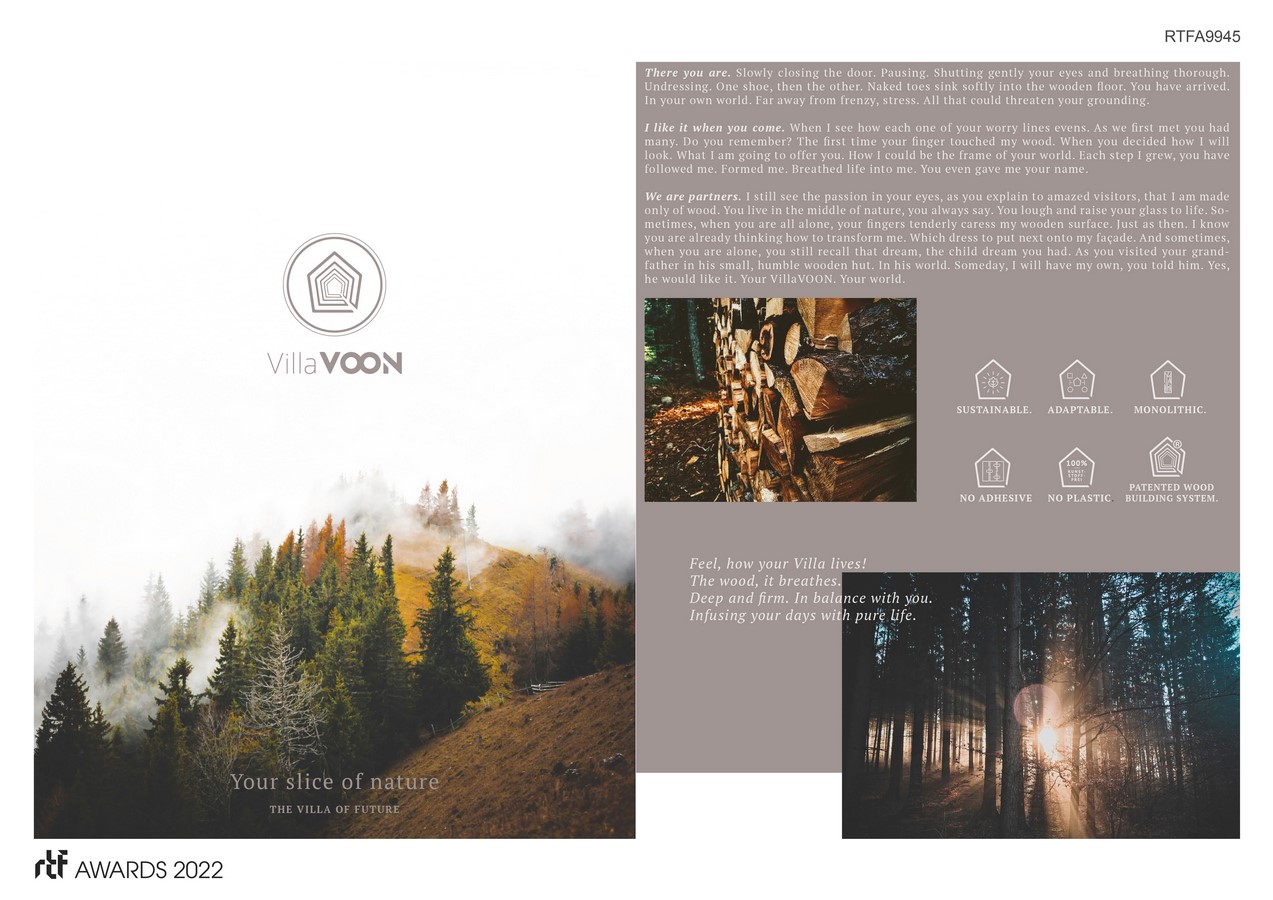This advertisement captures the allure of the award-winning getaway destination, Villavoon, which proudly boasts an "Awards 2022" accolade. Dominating the left side of the brochure, a large, captivating photograph showcases a stunning hillside adorned with tall pine and deciduous trees, the latter of which are in the midst of their beautiful autumn transformation. Amongst the trees and vibrant fall colors, a gentle mist envelops the hill, adding a mystical element to the scenery.

Above the hill picture, there is a small inset of a house icon set within a gray circle labeled "Villavoon." This image connects the serene landscape to the getaway location. On the right side of the brochure, complementing the main image, are two additional photographs: the first depicts rays of sunlight piercing through a grove of tall pine trees, illuminating the ground with warm, golden beams. The second image, positioned below, captures the cozy ambiance of a campfire or wooded campsite, ideal for a serene retreat into nature. Although the accompanying text is not readable, the rich imagery speaks volumes about the enchanting experience Villavoon offers.